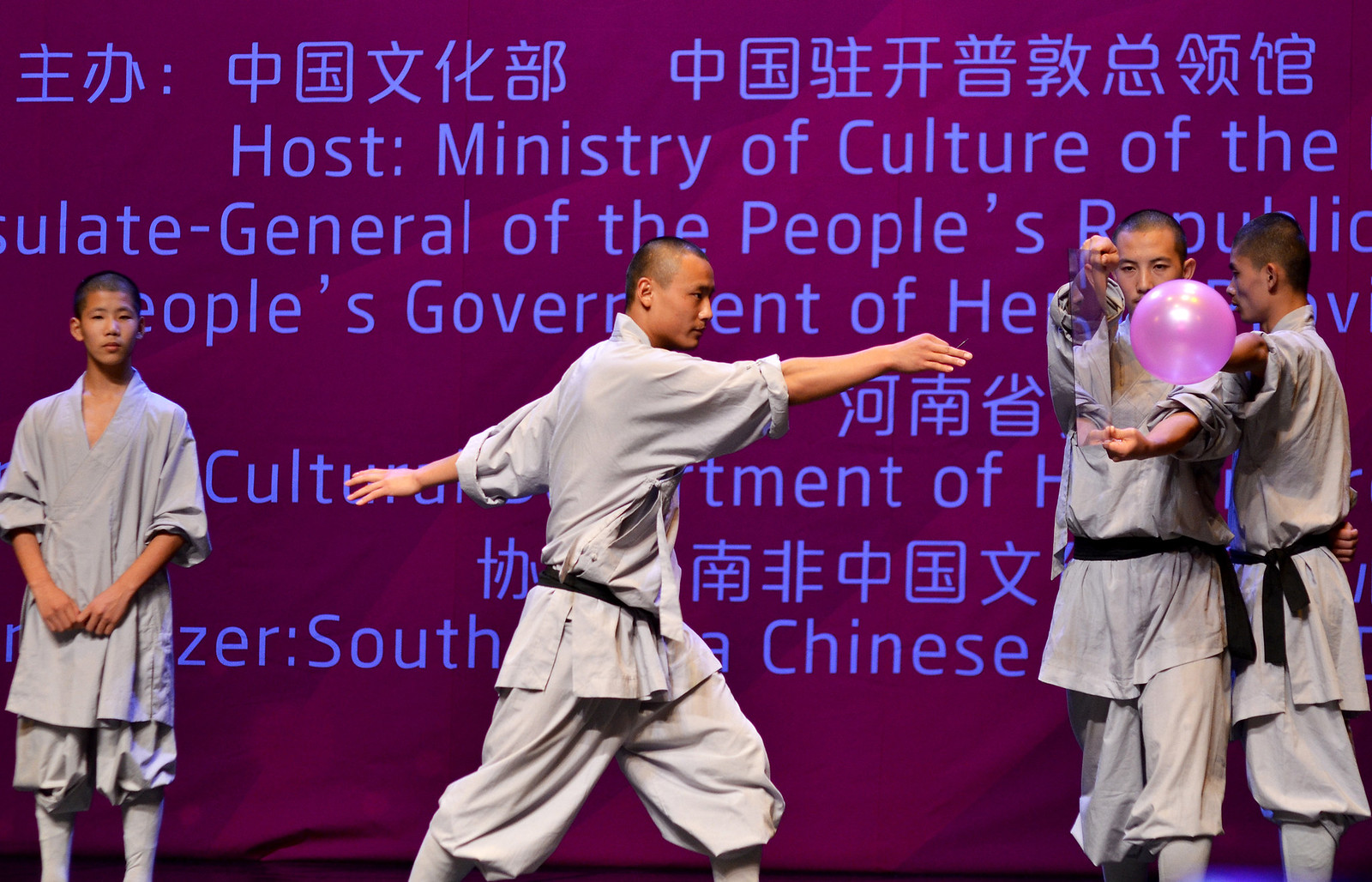The image depicts a group of Asian men on a stage, all donning traditional light gray karate uniforms, which consist of flowy robes or shirts paired with pants, and three of them are secured by black belts around their waists. Each man has short, dark hair, seemingly styled in a buzz or brush cut. On the far left, there's a man with a young boy, who is also dressed in a similar gray uniform, observing the scene. In the middle of the stage, one man stands with his arms outstretched, while to his side, another man appears to be performing a delicate manipulation of a pink balloon using a mirror held between his hands. The setup is illuminated by overhead spotlights, highlighting their facial features. They are performing in front of a large red or purple curtain that bears a partial inscription in white font, mentioning something about the "host Ministry of Culture" and "General of the People's Republic" in what appears to be a Chinese government event.